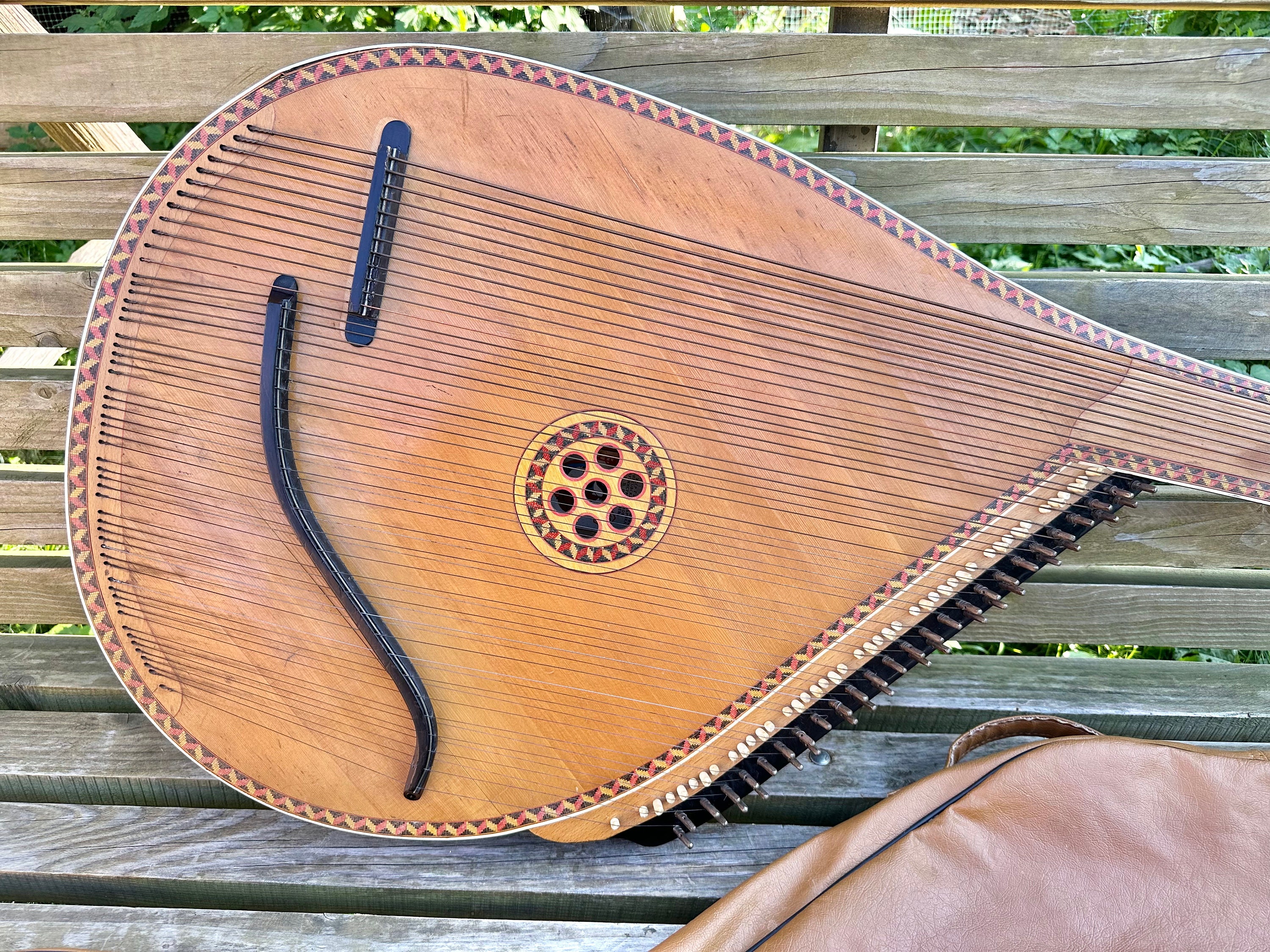In the photograph, the focal point is a wooden picnic bench set against a backdrop of lush greenery and trees. Resting on the bench is a uniquely intricate musical instrument, which seems to be a mandolin or guitar-like object characterized by its multitude of strings—potentially made from nylon or a composite material. The instrument itself is primarily light brown, accented with dark gray and orange zigzag patterns along the edges. A prominent circular design adorns the center of the instrument, surrounded by yellow and orange trims and featuring several small, red and black holes for sound resonance. This central design is a distinguishing feature, with an outer circle housing an intricate, smaller circular pattern. The instrument also includes a swirling black component at the top and is outlined with blue, red, and yellow hues in its detailed craftsmanship. Additionally, a brown leather purse is visible on the bench beside the instrument, contributing to the scene's rustic and casual outdoor setting.